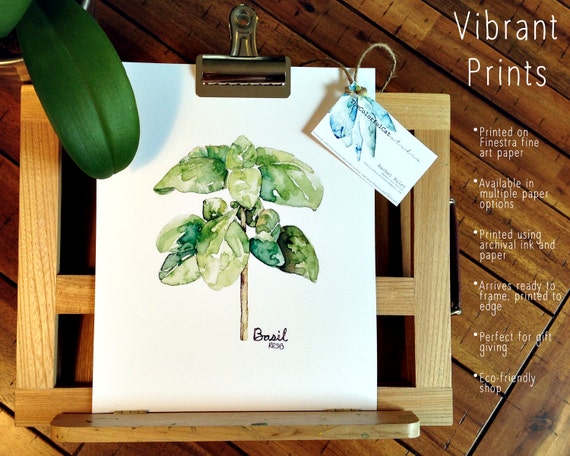The advertisement image prominently features a beautifully detailed watercolor painting of a basil plant, with leaves in varying shades of green from light to dark, some tinged with blue-green and gray. This painting is clipped at the top to a wooden artist's easel, standing against a backdrop of medium brown wooden slats. To the left of the easel, a smooth green leaf – possibly from an orchid – casts a soft shadow over the painting and easel. Attached to the painting with twine is a business card, predominantly white with blue watercolor accents, bearing the name "The Colorful Cat." Adjacent to the painting, a series of promotional bullet points presented in elegant text highlights the features of the print: "Vibrant Prints," "The First One Printed on Finestra Fine Art Paper," "Available in Multiple Paper Options," "Printed Using Archival Ink and Paper," "Arrives Ready to Frame," "Printed to Edge," "Perfect for All Giving," and "Eco-Friendly Shop." This carefully arranged image seamlessly blends artistic beauty with marketing information, situated on what seems to be a wooden floor or table.